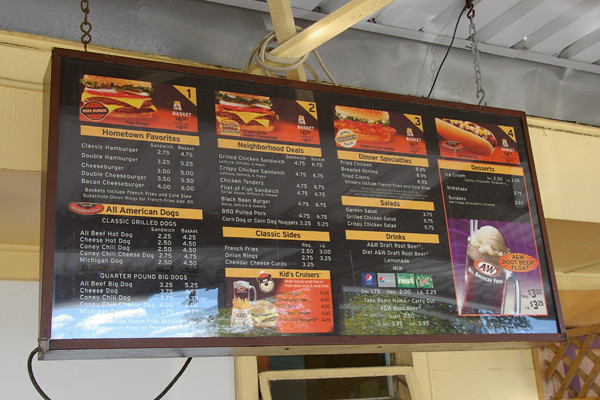This image is a vivid snapshot of an illuminated sign hanging inside a fast food restaurant. The environment suggests a casual, possibly franchise establishment, which serves A&W Root Beer, as indicated by the mention in the bottom right corner of the sign. The background reveals the underside of a metal roof, composed of white trough-like planks, alluding to a building with a metal frame structure. The upper part of the wall behind the sign is painted a pale yellow.

The sign itself is suspended from the ceiling by chains attached with S-hooks, and an electrical cord is visible running from the bottom left corner of the sign. It is framed in a dark wood-tone, but likely made of metal. The signage is electrified, probably with an acrylic lens illuminated by fluorescent or other lighting mechanisms.

The sign is divided into multiple sections with various menu items:

- The left-hand column is labeled "Hometown Favorites" and "All-American Dogs," featuring Classic Grilled Dogs, Beef, Coney Chili Dog, and other hot dog varieties. Though not fully legible, this section also seems to include various burgers.
- Across the top of the sign are combo meal options numbered 1 through 4. Combo 1 appears to be a cheeseburger combo, followed by another cheeseburger combo, a hamburger combo without cheese, and finally, a hot dog combo.
- The next section is "Neighborhood Deals," which presumably includes items like grilled chicken, although details aren't clear.
- The "Classic Sides" section lists options such as french fries, onion rings, and other sides not fully discernible in the image.
- The "Kid's Cruisers" section features a children's menu, adorned with a cartoon bear face.
- Following is "Dinner Specialties, Salads, and Drinks," although the specifics are difficult to make out.
- The final column showcases "Desserts," prominently featuring a root beer float.

Overall, the sign aims to highlight a variety of menu offerings, underscored by the classic presentation and nostalgic references, such as the A&W Root Beer float.